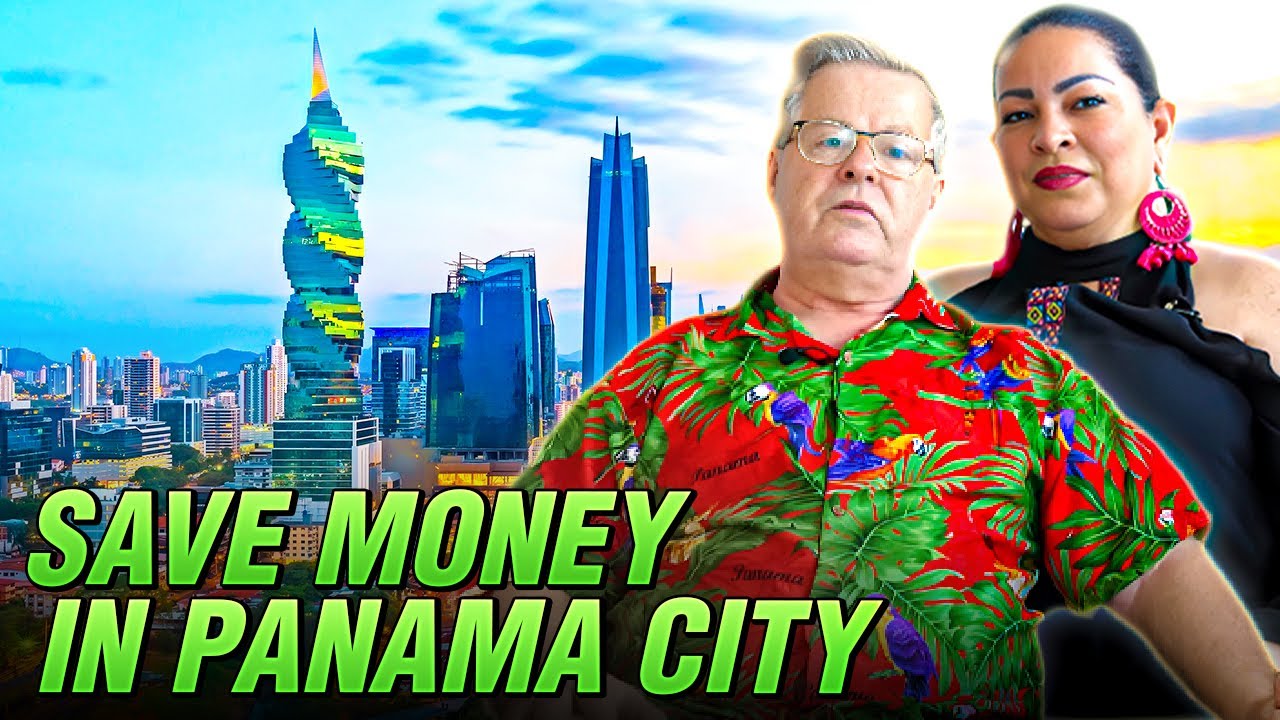The image portrays a vibrant website with a visually striking background. At the top, a blue sky transitions into deeper shades of blue adorned with fluffy white clouds. Touches of yellow and light purple streaks add a surreal dimension to the scene. As your eyes move downward, the skyline comes into view, featuring tall buildings shadowed in darker blues, likely reflecting the sky's hues. Among them, a distinctive, swirling skyscraper with glass windows stands out, its spiral form tapering to a point, mirroring the sky’s colorful reflections.

In the foreground on the right-hand side, a woman with dark, pulled-back hair and olive skin—suggestive of Latin heritage—adds a personal touch to the image. She wears striking long, pink circular earrings and red lipstick. Her outfit features a neckline that clasps around her neck, leaving her shoulders exposed. 

Adjacent to her, a heavyset man with graying hair and pale skin is seen wearing glasses. His attire consists of a vibrant red shirt, decorated with images of leaves, blue and yellow parrots, and emblazoned with the names of various cities, including Panama.

On the bottom left of the foreground, a bold green message says, "Save Money in Panama City," emphasizing the website's likely focus on budget-friendly travel or living.